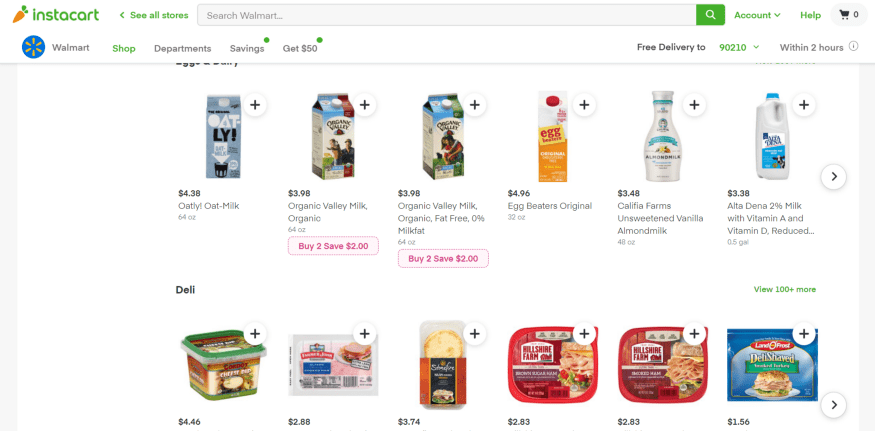This image is a screenshot of an Instacart shopping interface, featuring a white background. In the upper left-hand corner, the Instacart name and logo are displayed. The logo consists of the word "Instacart" written in green, alongside a simple illustration of an orange carrot. The section highlighted in this screenshot pertains to Wal-Mart, indicating that users can shop from Wal-Mart via Instacart for home delivery.

To the right of the Instacart logo, the Wal-Mart logo is prominently featured. This logo consists of a stylized blue circle with orange lines radiating outward, resembling rays of the sun. The top menu is visible, with options listed from left to right as follows: Shop, Departments, Savings, Get $50. On the right side of the menu, there is an informational snippet: "Free delivery to zip code 90210 within two hours."

The main content of the screenshot is divided into two rows of items. The top row shows different types of milk, including Oatly, Organic Valley Milk, Organic Valley Organic Fat-Free Milk, and Califia Farms Unsweetened Vanilla Almond Milk. The bottom row, labeled as the deli department, features various cuts of meat and other deli items. On the right side, there is a product from Land O' Lakes labeled "Deli Shaved." To the left of that is an item from Hillshire Farm, along with some cheese. Each item is accompanied by an image to help users identify the products.